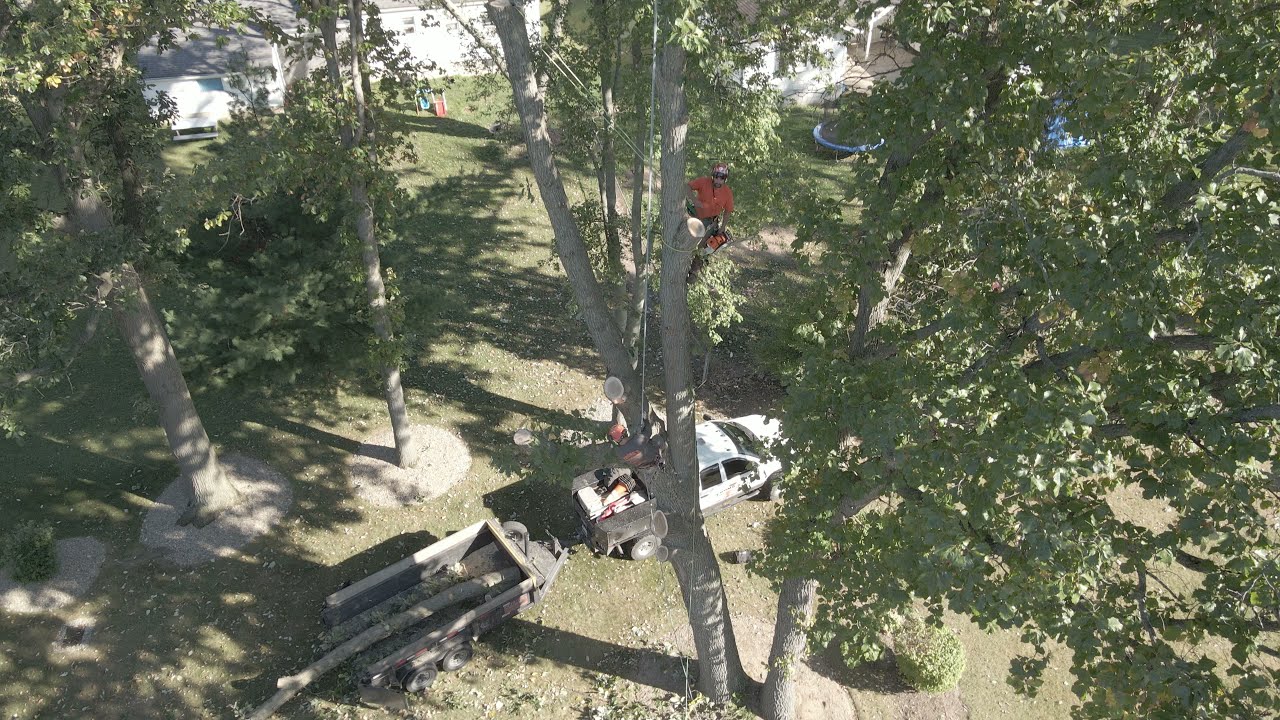In this image, a tree trimmer is meticulously working high up in a large tree, approximately 75 feet above the ground, in what appears to be a spacious front yard of a white-painted house. The man, clad in an orange t-shirt and a metal helmet with a face guard, is securely fastened by a rope around his waist, which is tied to a sturdy limb. He is wielding an orange chainsaw as he cuts down substantial branches. Two large cut branches already lie in a trailer hitched to a white truck at the base of the tree. The scene is dominated by the vibrant green leaves of the trees, with various elements like trampolines and parts of other houses visible in the background. The expansive yard and clear weather hint at a leisurely, suburban setting, enriched with shades of green, blue, white, red, and brown, painting a vivid picture of a professional at work in what seems to be a residential area.